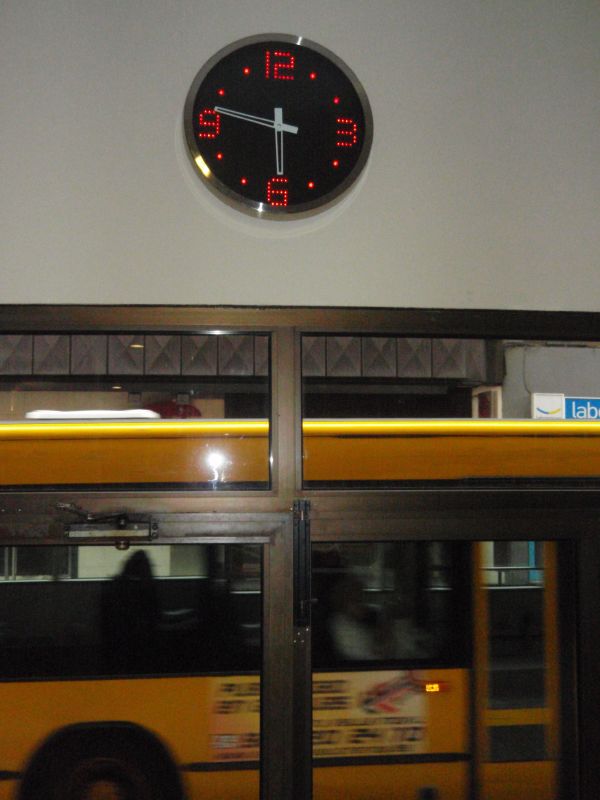This photograph captures a dynamic scene featuring a black-faced clock with red digital numbers displaying the time as approximately 6:46. The clock is mounted above a doorway that appears to lead outside. The face of the clock prominently displays the numbers 12, 3, 6, and 9, with dots marking the other hours. Through the doorway, a large yellow bus zooms past, creating a noticeable motion blur. The bus partially obscures a sign, rendering it unreadable as it moves behind a post that separates the doorway from an adjacent window. Above the door and the larger window to the right are smaller rectangular windows, adding architectural detail. The dark brown metal door frame contrasts with the outdoor light. Additionally, a sign above the bus and the facade of a building across the street are faintly visible, providing context to the location's urban setting.